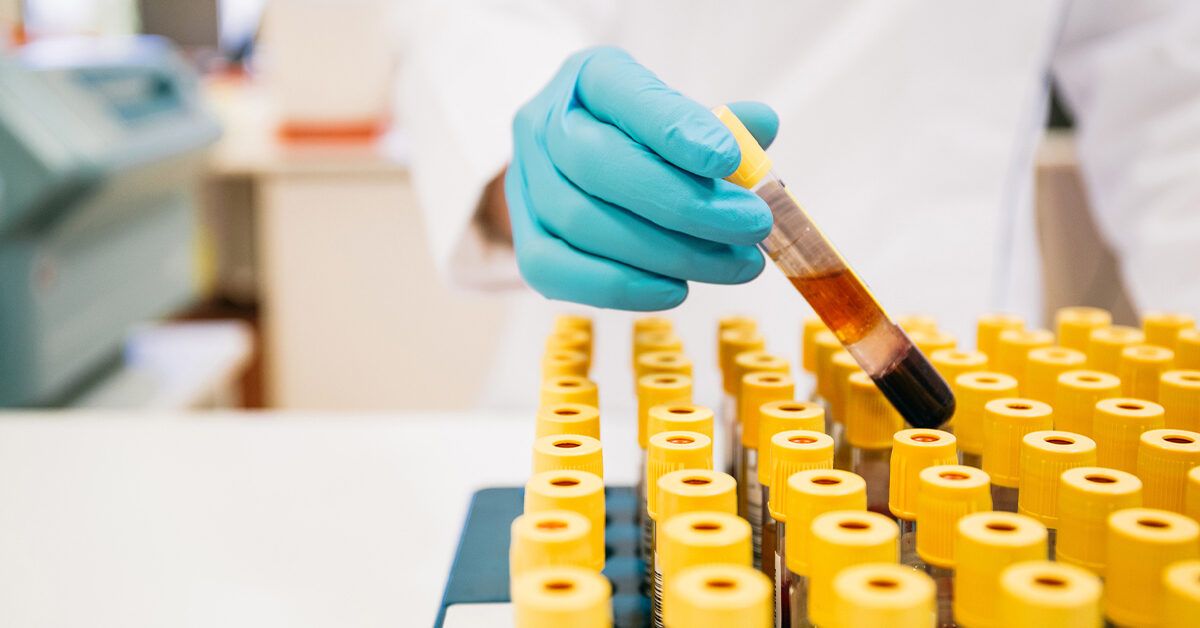In this detailed indoor photograph, a medical technician or lab worker, easily identified by their green gloves and white lab coat, is carefully extracting a test tube with a yellow cap from a tray of identical tubes arranged in neat rows on a white countertop. The test tube seems to contain a mix of liquids, with the top part appearing clear, the middle orange, and the bottom dark brown, possibly blood. The technician's gloved hand and the vials on the countertop are in sharp focus, while the background remains blurred, featuring indistinct equipment that might be used for lab analyses, like a printer or a vial reader. This scene captures the meticulous nature of laboratory work, emphasizing the technician's precise handling within a clinical setting.